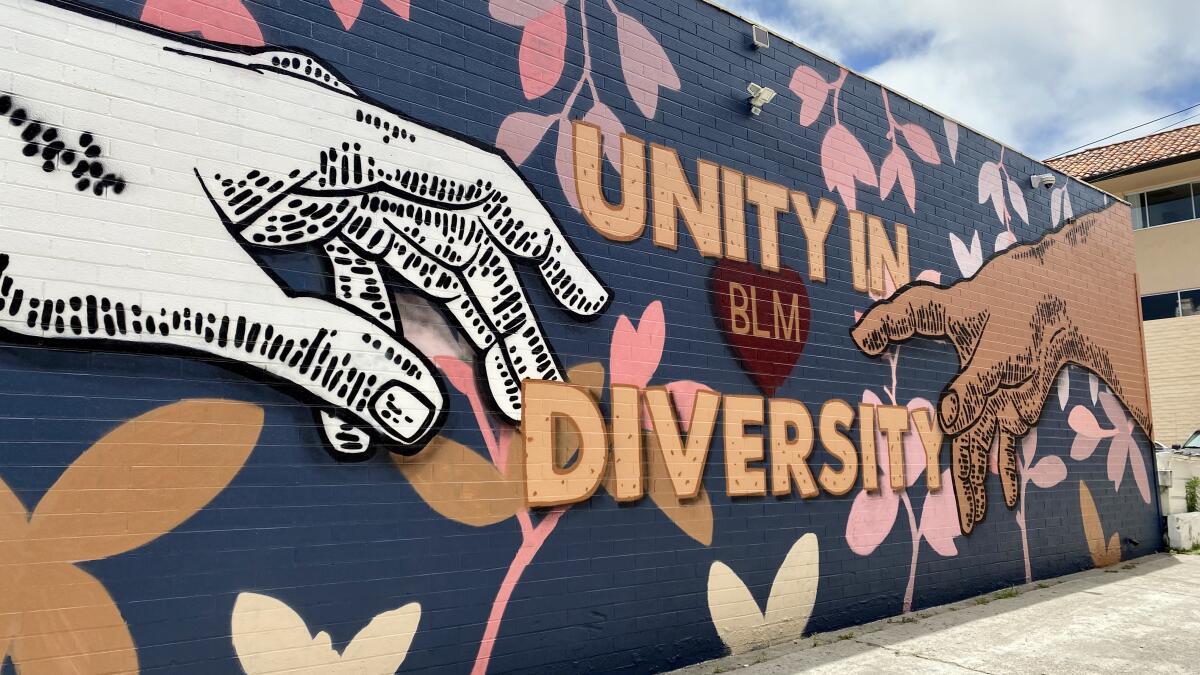This is a rectangular landscape photo of a street scene featuring a tall brick building adorned with a vibrant mural. The building's wall is covered in colorful graffiti with a deep bluish-gray background. Prominently displayed in large yellow block lettering are the words "Unity in Diversity," with a red heart in the center containing the letters "BLM" in yellow. Flanking the heart, two stylized hands reach towards each other—one on the left is white, and the other on the right is brown, both detailed with black lines to indicate texture. Surrounding the text and hands, the mural is decorated with flower petals in shades of pink, white, orange, tan, and lilac. The building stands on a concrete street, and the background reveals another building and a blue sky with white clouds.